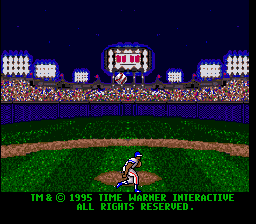A vibrant color photograph captures a nostalgic video game scene from 1995, with fluorescent green text at the bottom reading "TM and copyright 1995, Time Warner Interactive, all rights reserved" against a black background. The image presents a classic baseball video game with a detailed depiction of a baseball field from a third-person perspective. Centrally located on the pitcher's mound is a player, donned in a white uniform accented with red and blue trim, complemented by a black helmet or cap and blue shoes. The player is poised to pitch, facing to the right. Above him, a baseball is suspended mid-air, with a trail of motion dots indicating its past trajectory. In the background, pixelated fans fill the stands, portrayed by dotted patterns that span horizontally. The stadium's lighting is represented by six large square structures positioned symmetrically—three on each side of the screen—each composed of smaller squares arranged in a grid pattern. Dominating the center of the background is a pixelated scoreboard, a hallmark of the retro gaming experience.